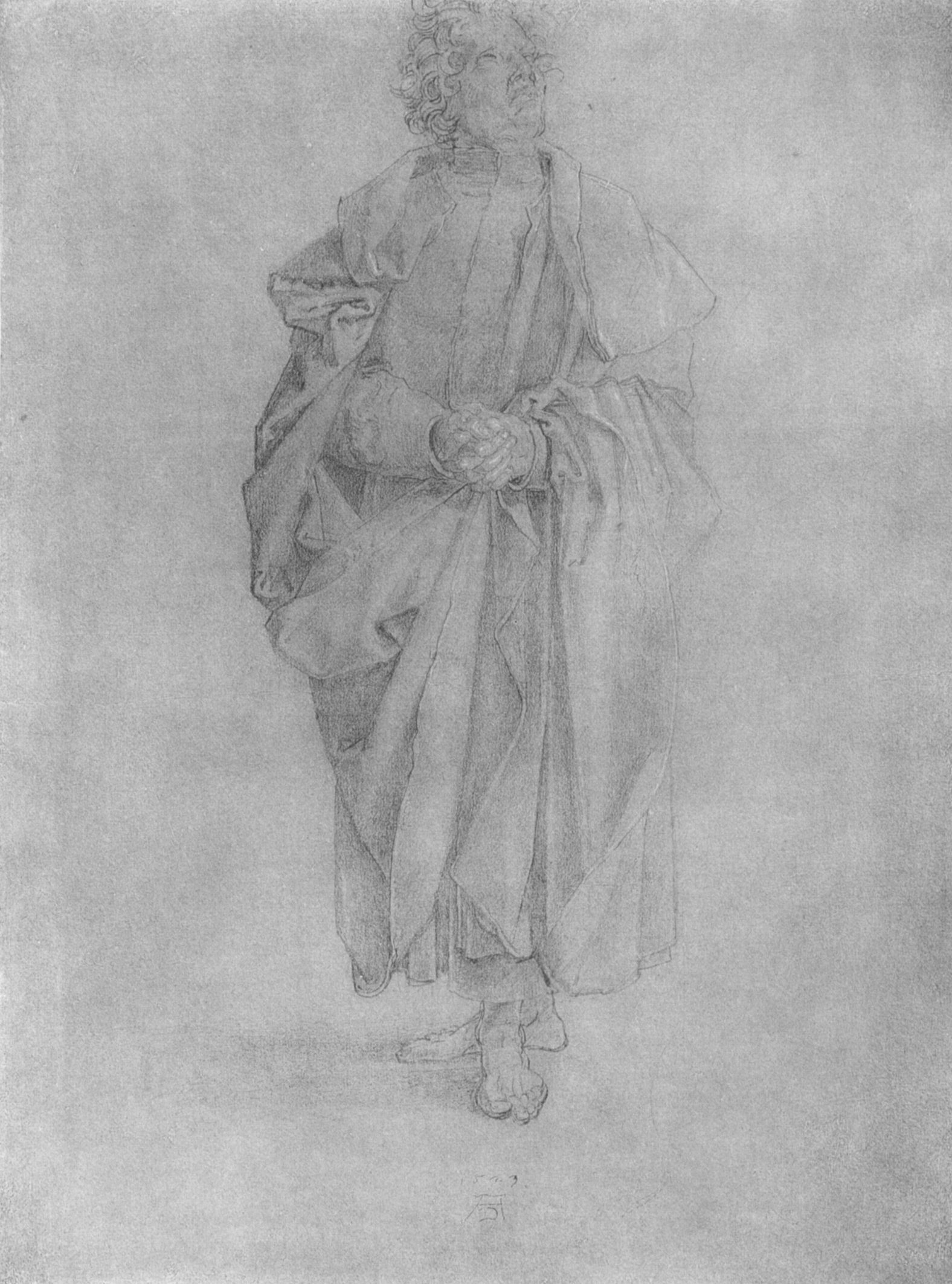This hand-sketched, black and white drawing features a man from medieval times and is characterized by its dim tones and lack of intense detail. The man, with curly, chin-length hair and a serious expression, is barefoot and stands with his left foot forward and his right foot slightly braced behind. He is dressed in an ornate, layered robe with abundant folds and creases that flow down from his shoulders to just above his ankles. The robe, starting like a frock and forming a thick collar around the shoulders, has sleeves extending down to his wrists. He clasps his hands tightly in front of him and gazes upwards and to the left into a vast, empty space, evoking a somber, contemplative atmosphere.